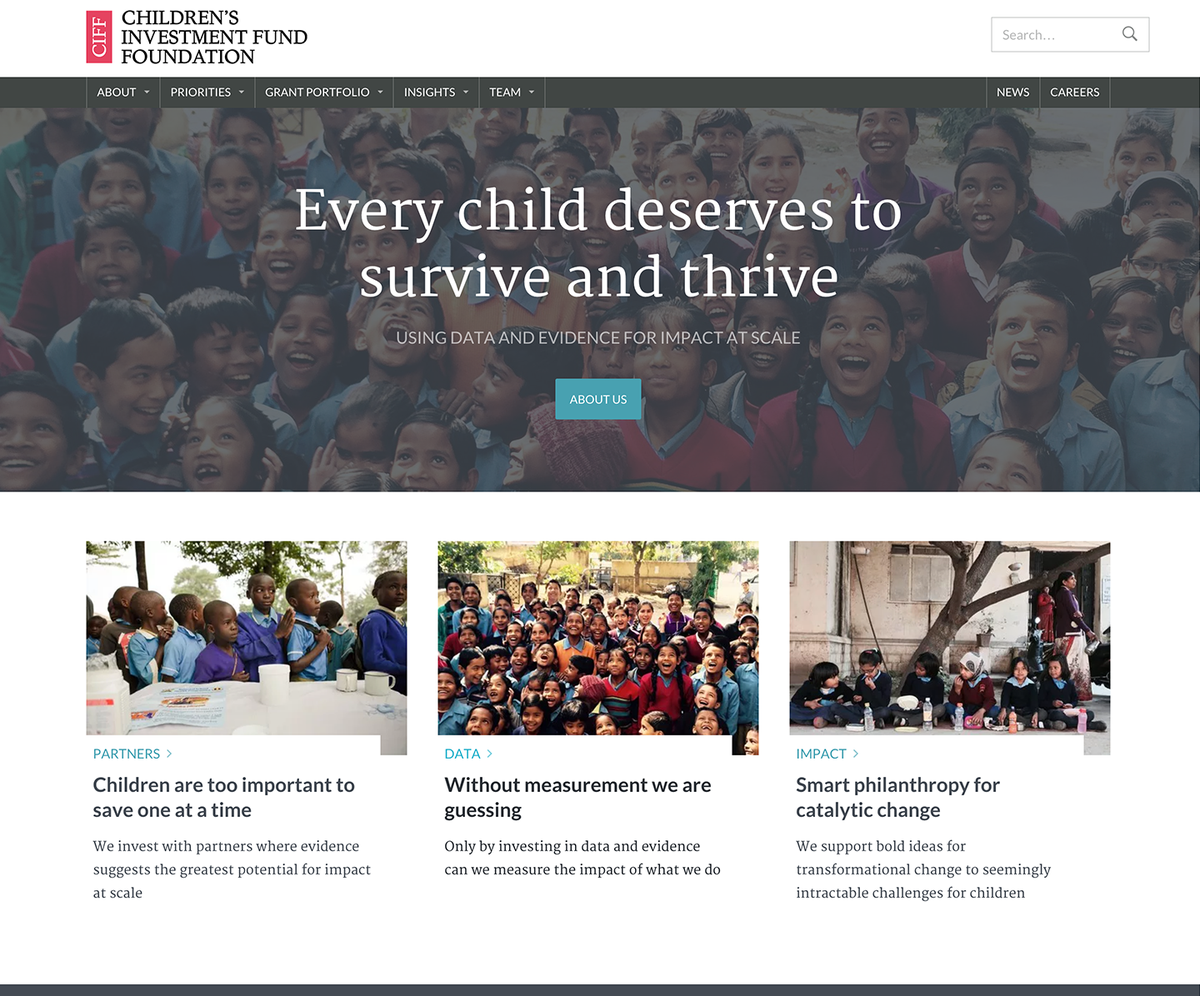This image appears to be a screenshot of the homepage of the Children's Investment Fund Foundation (CIFF) website. In the upper left corner, the CIFF logo is visible, featuring a rectangular shape with a red background. Directly below the logo is a dark gray horizontal menu bar, containing several clickable links labeled: About, Priorities, Grand Portfolio, Insight, and Team. On the far right of the same menu bar, additional links titled News and Careers are displayed in white text.

Above the menu bar, there's a light gray bordered search bar with a white background, complemented by a magnifying glass icon on the right side for search functionality. 

Dominating the central area of the homepage is a wide, rectangular photograph depicting a group of smiling and happy children looking upwards, conveying a sense of joy and enthusiasm. Superimposed on this image is a white text message that reads: "Every Child Deserves to Survive and Thrive." Below this headline, a blue rectangular button with white text entices users to learn more with its label: About Us.

Beneath the main photograph, there are three article previews, each represented by a rectangular image featuring groups of children. These preview images serve as visual teasers for the content, likely focusing on various initiatives and stories related to the foundation's mission and activities.